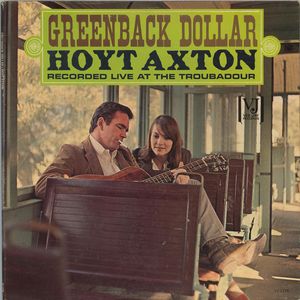The album art for Greenback Dollar's "Hoyt Axton: Recorded Live at the Troubadour" features a detailed, sepia-toned painting set inside a classic train carriage. The scene is richly depicted with brown train seats arranged in rows. At the center, a white man with brown hair, dressed in a brown suit jacket, white undershirt, and brown cowboy boots, plays a guitar with a cigarette hanging from his mouth. Behind him, a white brunette woman wearing a black jacket and white blouse sits in another seat, gazing intently at the guitarist. The background includes windows with green trim, enhancing the rustic ambiance, while the benches have slats and are colored in muted tones. Above this evocative scene, the album's title and artist are displayed prominently in a green rectangular box with pea green circles: "Greenback Dollar" in large brown uppercase letters, "Hoyt Axton" in smaller black font, and "Recorded Live at the Troubadour" in even smaller black letters below. The overall imagery captures a nostalgic and intimate atmosphere.